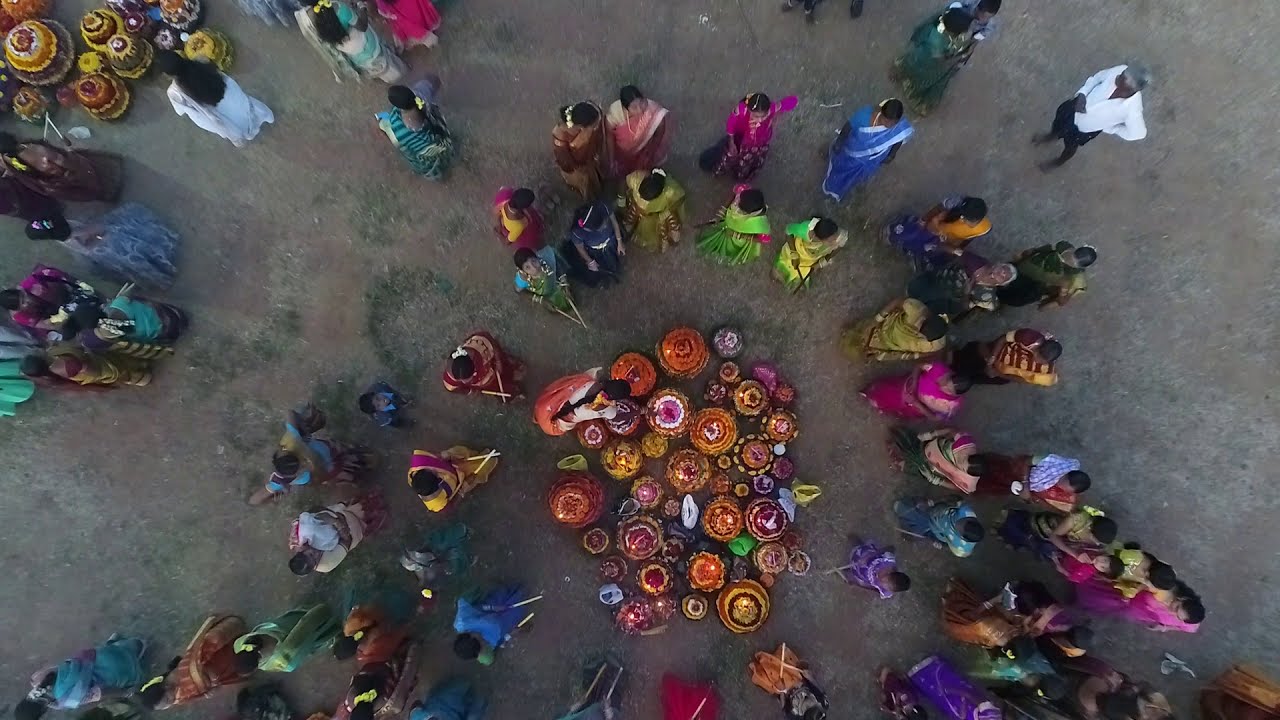This overhead image captures the lively scene of an Indian festival. The focal point is a series of colorful, circular woven baskets with lids, around which a large group of people has gathered in a circle. The ground is relatively flat with sparse patches of vegetation. The participants, predominantly women dressed in vibrant saris of blues, greens, pinks, and yellows, add splashes of color to the scene. Many of these women hold what appear to be drum sticks, indicating that a musical performance might be imminent. A few men are present, distinguished by their white shirts and black pants. Another set of these baskets can be seen in the top left corner of the image. The image appears to be set on a road or plaza, enhancing the communal atmosphere of this cultural celebration.